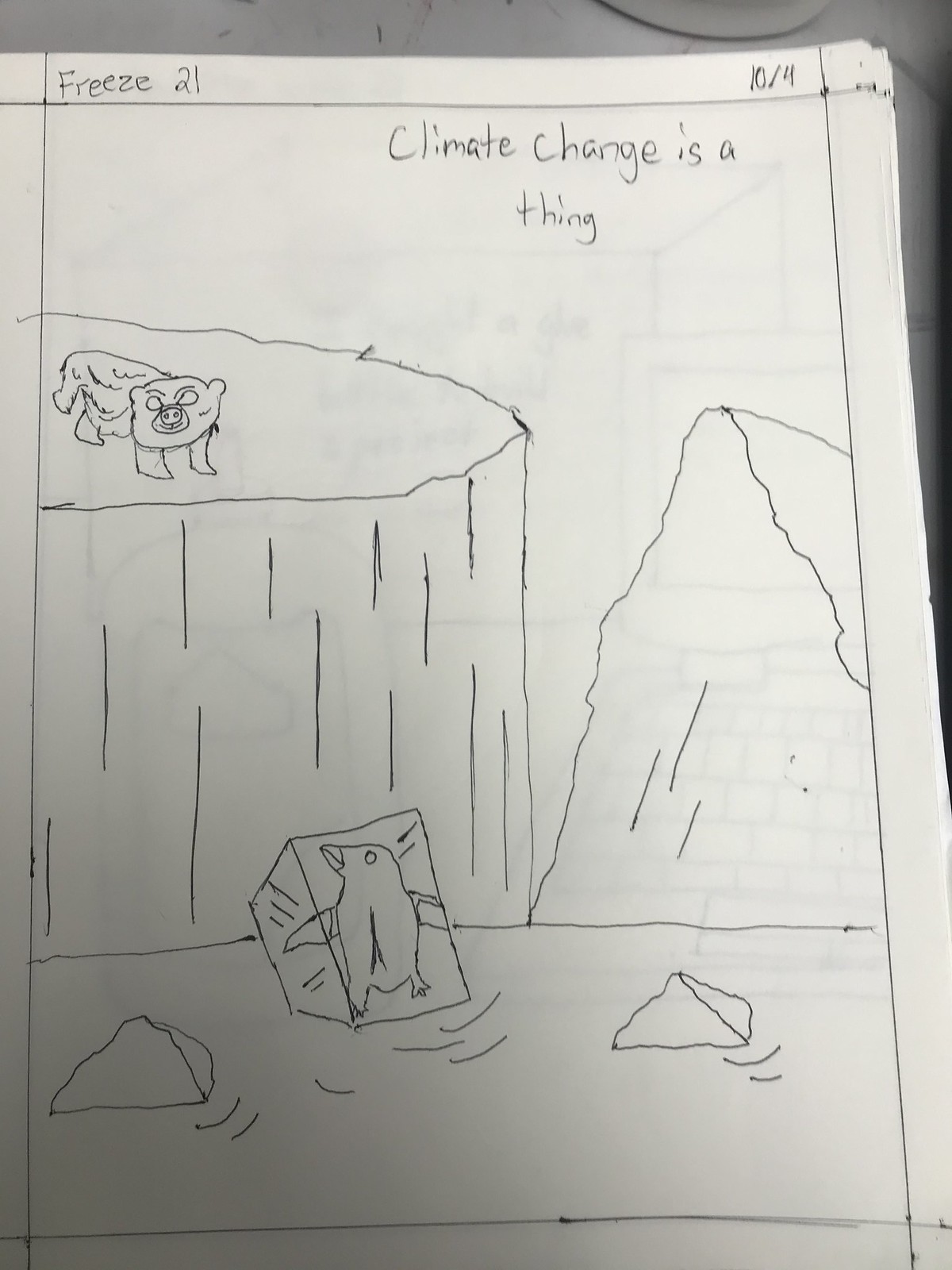The vertical rectangular drawing on white paper, apparently sketched with a pen, vividly depicts a scene relating to climate change. Titled "Climate Change is a Thing" at the top, with additional annotations such as "freeze 21" in the top left corner and "10/4" in the top right, the focal points of the drawing include an Arctic-like environment. At the bottom of the drawing, a small penguin is encased in a large ice cube, floating in a body of water surrounded by smaller ice chunks. To the left, atop a tall ice structure with vertical lines, stands a four-legged animal resembling a snow leopard or a bear, positioned horizontally and appearing vigilant. The entire scene, rendered meticulously in pen, conveys a stark message about the impacts of climate change on arctic wildlife and habitats.